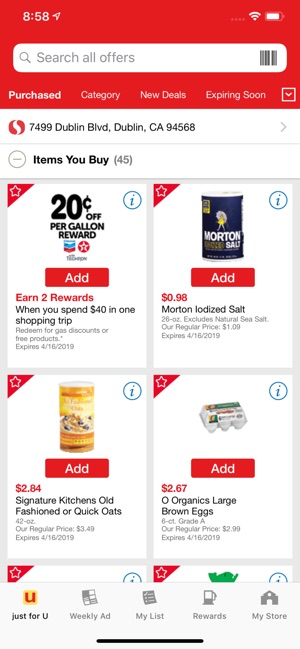Screenshot of a mobile device displaying an application interface. 

**Top Left:**
- Time: 8:58 

**Top Right:**
- Network signal bar: Blank (indicating no network or no SIM)
- WiFi signal icon: Visible 
- Battery level indicator: Visible 

**Below Status Bar:**
- Search field with placeholder text: "Search all offers, purchased, category, new deals, expiring soon"
- Location: "7499 Dublin Boulevard, Dublin, California 94568"

**Lower Section:**
- Summary of items purchased: "Items you buy: 45"
- Four visible items/offers listed:
  1. "20 cents off per gallon reward"
  2. "In-store rewards when you spend $40 on one shopping trip"